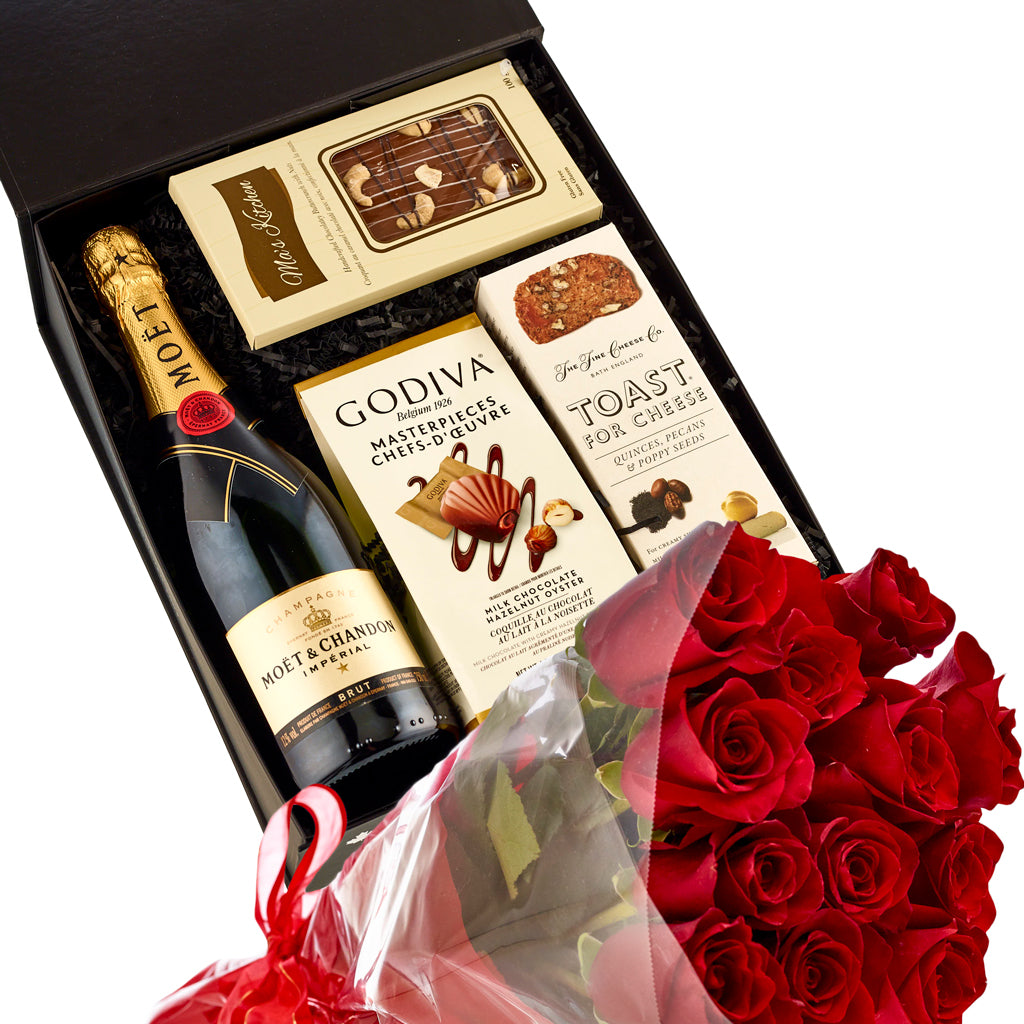The photograph features an open, black rectangular gift box filled with various luxurious items, perfect for a special occasion such as Valentine’s Day. The left side of the box contains a bottle of Moët & Chandon Imperial Champagne with its distinctive gold foil and red seal. Adjacent to the Champagne bottle on the right, there are two bars of chocolate; one can be identified as a thin rectangle with possible nuts on top. Below the chocolate bars, there is a bag of Godiva Masterpieces showcasing milk chocolate hazelnut oysters. Beside these treats, there is also a longer rectangular package labeled "Toast for Cheese," decorated with images of pecans and poppy seeds. Completing the ensemble, a bouquet of a dozen red roses wrapped in cellophane and adorned with a red and white ribbon lies below the gift box, enhancing the presentation with a romantic touch.